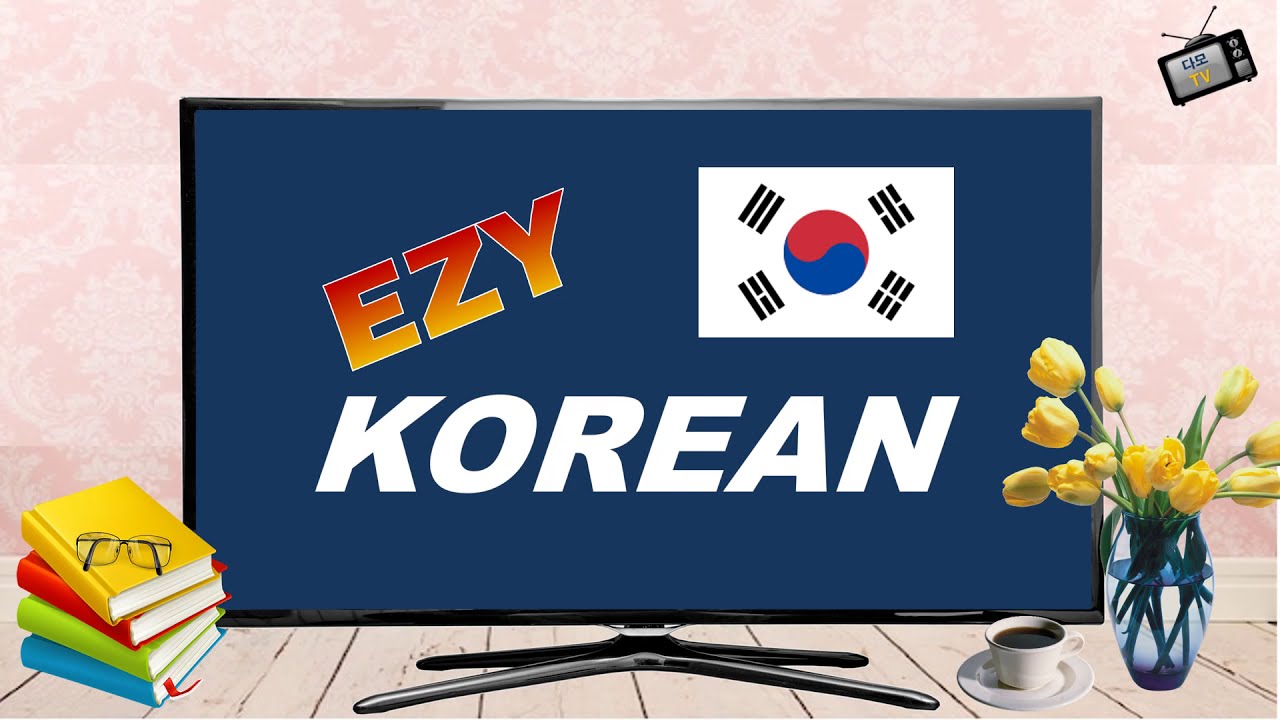The image depicts a stylized and somewhat abstract collage centered around a flat screen TV or computer monitor placed on a white wooden surface against a backdrop of pink and white wallpaper. The screen itself is predominantly blue, featuring the text "EZY" in bold red and yellow print tilted diagonally upwards, with "Korean" written below in a simpler font alongside a Korean flag. In the top right corner of the screen, there is a small icon resembling a tiny TV, displaying Asian characters followed by the word "TV" in yellow text. 

Adjacent to the TV, on the right, stands a glass vase containing yellow tulips, filled with water a little more than halfway. To the left of this vase, there's a white coffee cup filled with black coffee, resting on a matching saucer. To the far left of the TV, a stack of four books in blue, green, red, and yellow lies on the floor, topped with a pair of eyeglasses. The composition is rich in color, featuring shades of blue, red, yellow, green, pink, orange, and black, blending together to create an eye-catching advertisement, likely promoting an educational tool or TV program titled "Easy Korean."